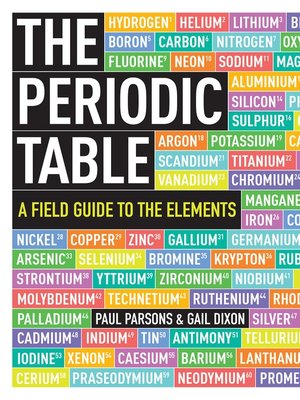This image shows an eye-catching cover, likely of a book or a poster, titled "The Periodic Table," with the subtitle "A Field Guide to the Elements." The prominent title is left-aligned, featuring large white text on a black background. The subtitle beneath it is in yellow, also set against a black background. Surrounding the title and subtitle are the names of all the elements from the periodic table, such as hydrogen, helium, lithium, boron, cesium, and palladium. These names are written in all caps within colorful rectangles of various bright colors, including orange, red, purple, blue, green, and teal, which repeat in a vibrant pattern. Toward the bottom center, the book lists its authors, Paul Parsons and Gail Dixon. The cover's striking, rainbow-like palette and educational content suggest it would be ideally suited for a school environment.